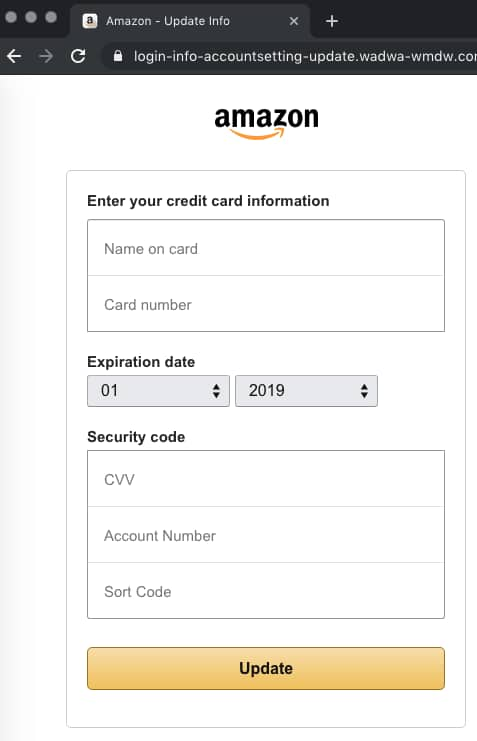Screenshot of an Amazon Payment Information Page on a Mobile Device

This screenshot captures a mobile interface of an Amazon payment information page. At the top, within a black rectangle with white text, are the navigation options: "Amazon-updateinfo, login-info-accountsetting-update." Below this header, prominently displayed is the Amazon logo: "Amazon" in black lettering with the iconic yellow arrow swooping from 'A' to 'Z'.

The main section invites users to "Enter your credit card information." This section is set against a black background with the instructions and fields in contrasting white. Two input boxes are provided with gray placeholder text: "Name on card" for entering the cardholder’s name and "Card number" for inputting the card number.

Below these, there are two dropdown boxes for the card's expiration date. The first dropdown, defaulted to "01," allows users to select the expiration month, while the second, preset to "2019," lets users choose the expiration year.

Further down, additional fields include "Security code" for the CVV, "Account number," and "Sort code," each within distinct rectangles.

At the bottom of the page is a yellow "Update" button with black text, prompting the user to confirm and save their payment information.